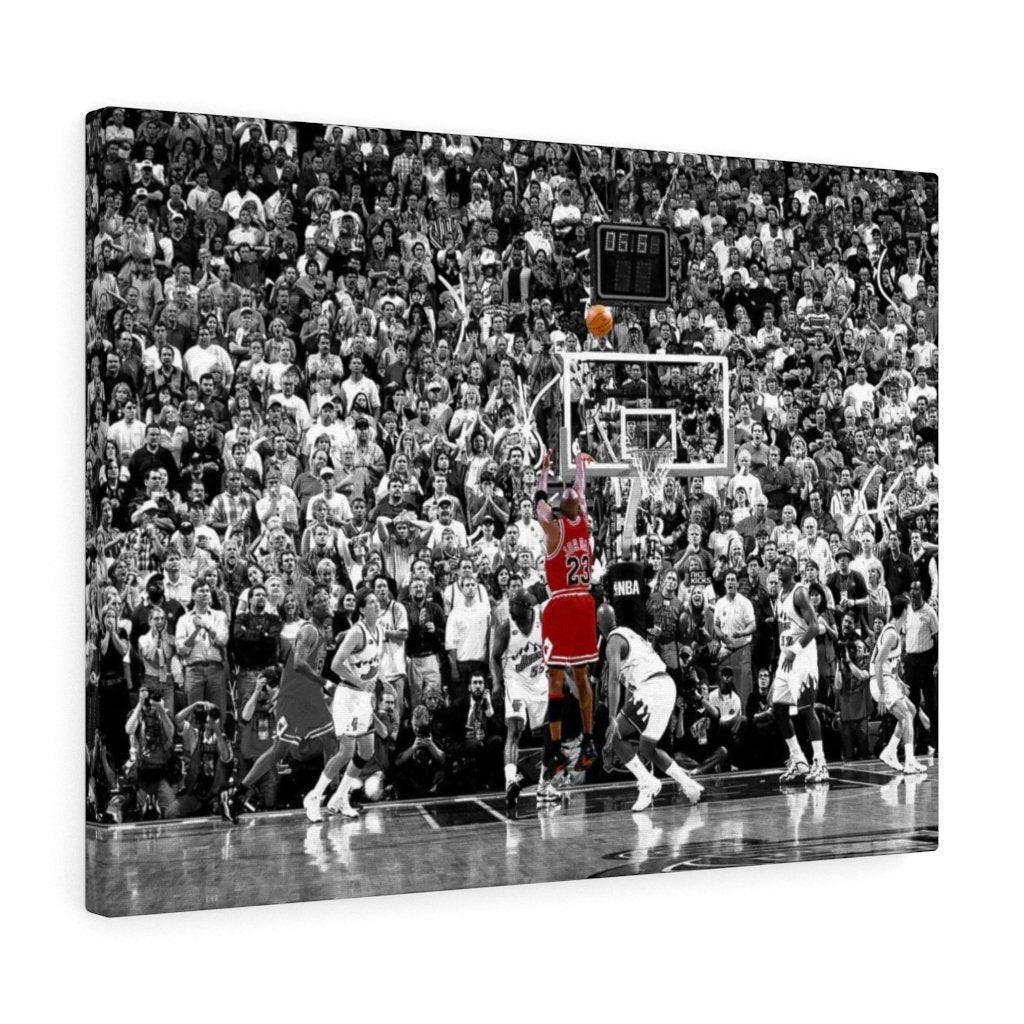This image is a striking canvas print of a memorable moment from the 1998 NBA Finals, featuring basketball legend Michael Jordan. The scene captures Jordan in mid-air, wearing his iconic red Chicago Bulls jersey and black shoes, having just released a shot. The ball, vividly orange, hangs in the air, midway between Jordan and the basket. The unique artistry of the image is highlighted by the black-and-white treatment of the background, which includes a mesmerized crowd and players from both the Chicago Bulls and the Utah Jazz—all rendered in grayscale. This artistic choice dramatically emphasizes Jordan in full color, drawing all attention to his poised, athletic form as he executes the game-winning shot. The canvas, designed for wall display, masterfully blends color alteration to focus on Michael Jordan, making it a standout piece that captures the intensity and significance of the pivotal moment in basketball history.